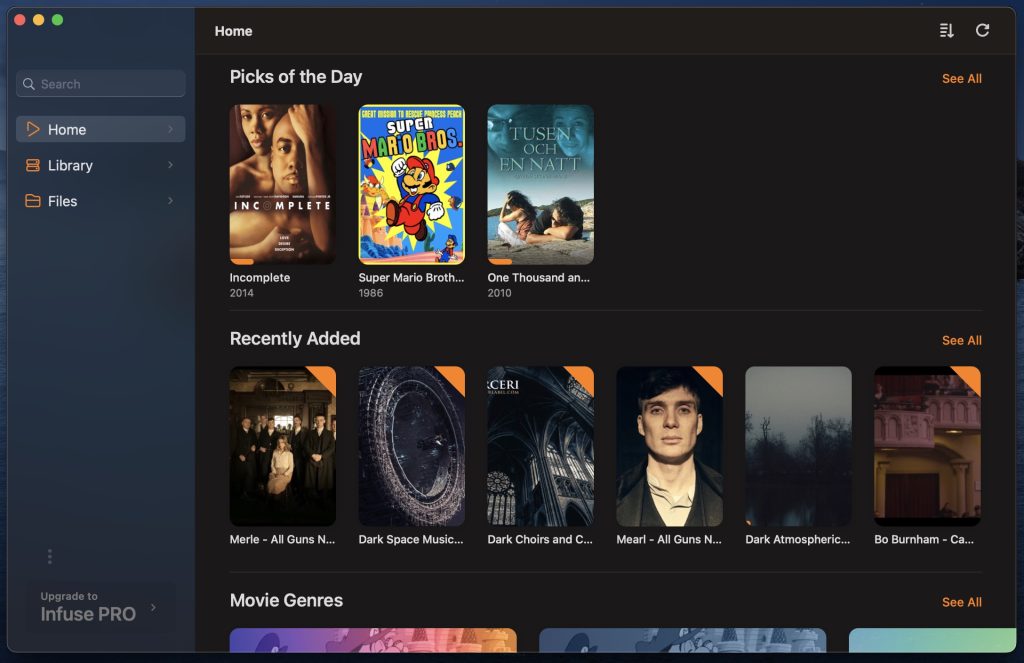**Screenshot Description: Infuse App Interface**

The screenshot showcases the user interface of the Infuse application with a black background. The left sidebar features a slightly different shade of black and contains several navigation and action buttons:

1. **Top Left Corner**:
   - **Traffic Light Icons**: Three colored dots (red, yellow, green) in the top-left corner.
   - **Search Box**: Below the dots, a light gray search area is present, highlighted with a white magnifying glass icon and the word "Search" in capital letters.

2. **Navigation Menu**:
   - **Home**: Highlighted in light gray, with an orange arrow pointing to the right and the word "Home" in white with a capital H.
   - **Libraries**: Below Home, shown as two orange-bordered books stacked with a black fill, accompanied by an orange right-arrow and the word "Libraries" in white with a capital L.
   - **Files**: Finally, a folder icon with an orange border and black fill, also with an orange right-arrow and the word "Files" in white with a capital F.

3. **Upgrade Section**:
   - At the bottom of the sidebar, the text "Upgrade to Infuse Pro" is displayed in capital letters, with an arrow pointing to the right. Above it, three gray dots.

4. **Main Interface**:
   - **Top Navigation**:
     - The top of the main section is marked by a thin black header.
     - On the right side, four horizontal lines with a down-arrow next to them, a refresh icon to their right.
   - **Content Area**:
     - **Header**: "Home" is written in white with a capital H.
     - **Featured Section**:
       - **Pics of the Day**: Written in capital letters and white font.
       - **Advertisements**:
         - **Incomplete (2014)**: Featuring an African-American couple.
         - **Super Mario Brothers (1986)**: An image of Mario jumping with a yellow sun backdrop.
         - **1000 ... (2010)**: Film or media advertisement.

5. **Recently Added**:
   - **Section Header**: "Recently Added" in white capital letters, marked by a dark gray separator line, and a "See All" option on the top right.
   - **Content Thumbnails**:
     - **Merle - All Guns N ...**: Multiple entries with gray backgrounds, images ranging from a tire (Dark Space Music) to a cathedral (Dark Choirs), with relevant titles and incomplete text.
     - **Bo Burnham - CA ...**: A building façade with pink bricks, showing part of the title with an orange corner mark.
     - **Movie Genres**: Additional section header in white, capital letters, with further thumbnails partially visible beneath it.

This comprehensive interface captures an organized structure with distinct navigation, upgrade options, and curated content areas suitable for a multimedia application.